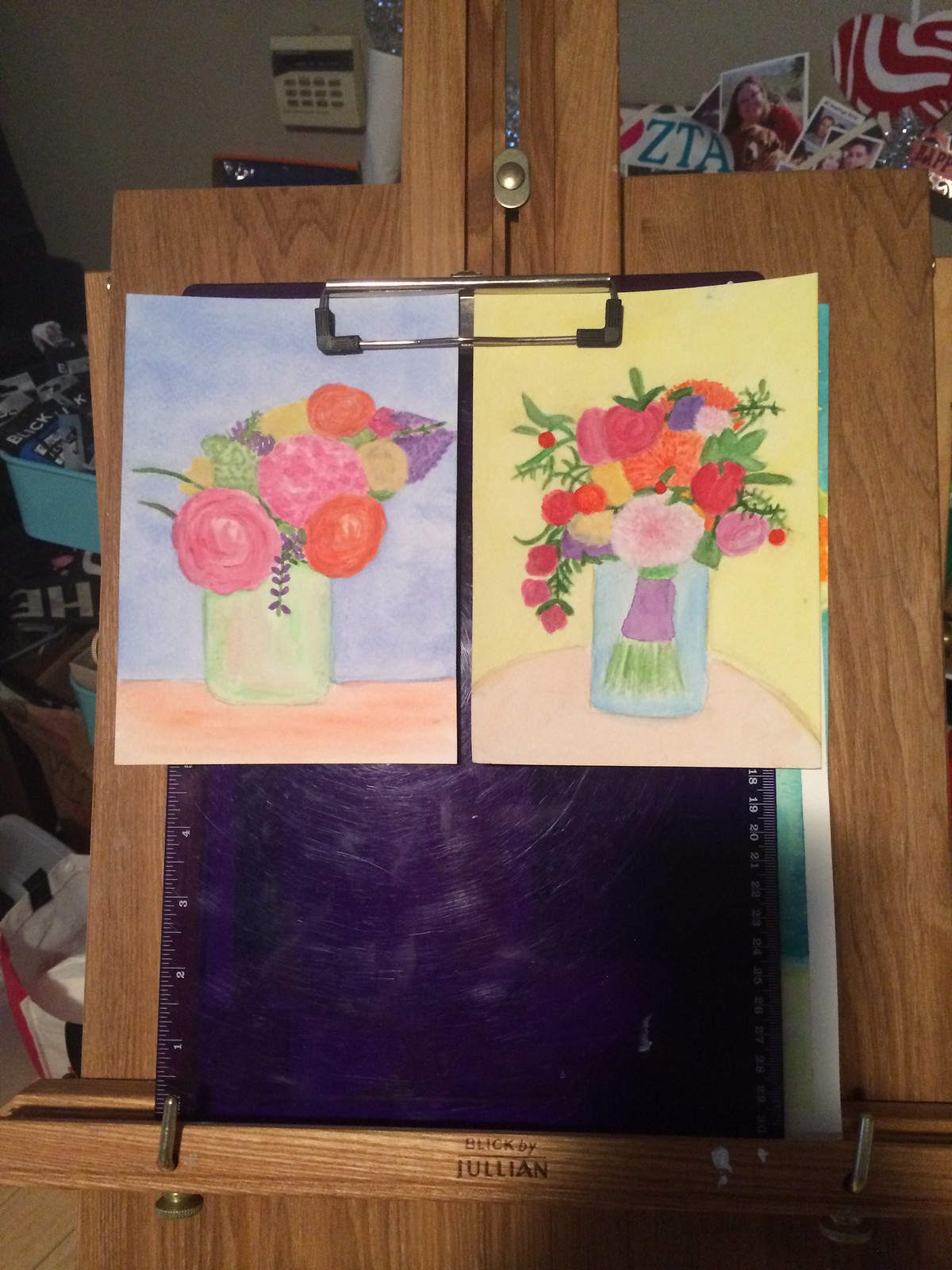The image features a vibrant purple clipboard holding two pieces of artwork, both depicting flowers and plants in pots. The clipboard has a silver and black clip at the top, securing the artworks in place. The surface behind the clipboard is brown. Central to the surface below the clipboard, the text reads "BLIK" in uppercase letters, spelled B-L-I-K, and underneath it reads "JULIAN," spelled J-U-L-I-A-N. The overall scene is well-composed, highlighting the artistic representations and the vivid colors of the clipboard, contrasting elegantly with the brown background.